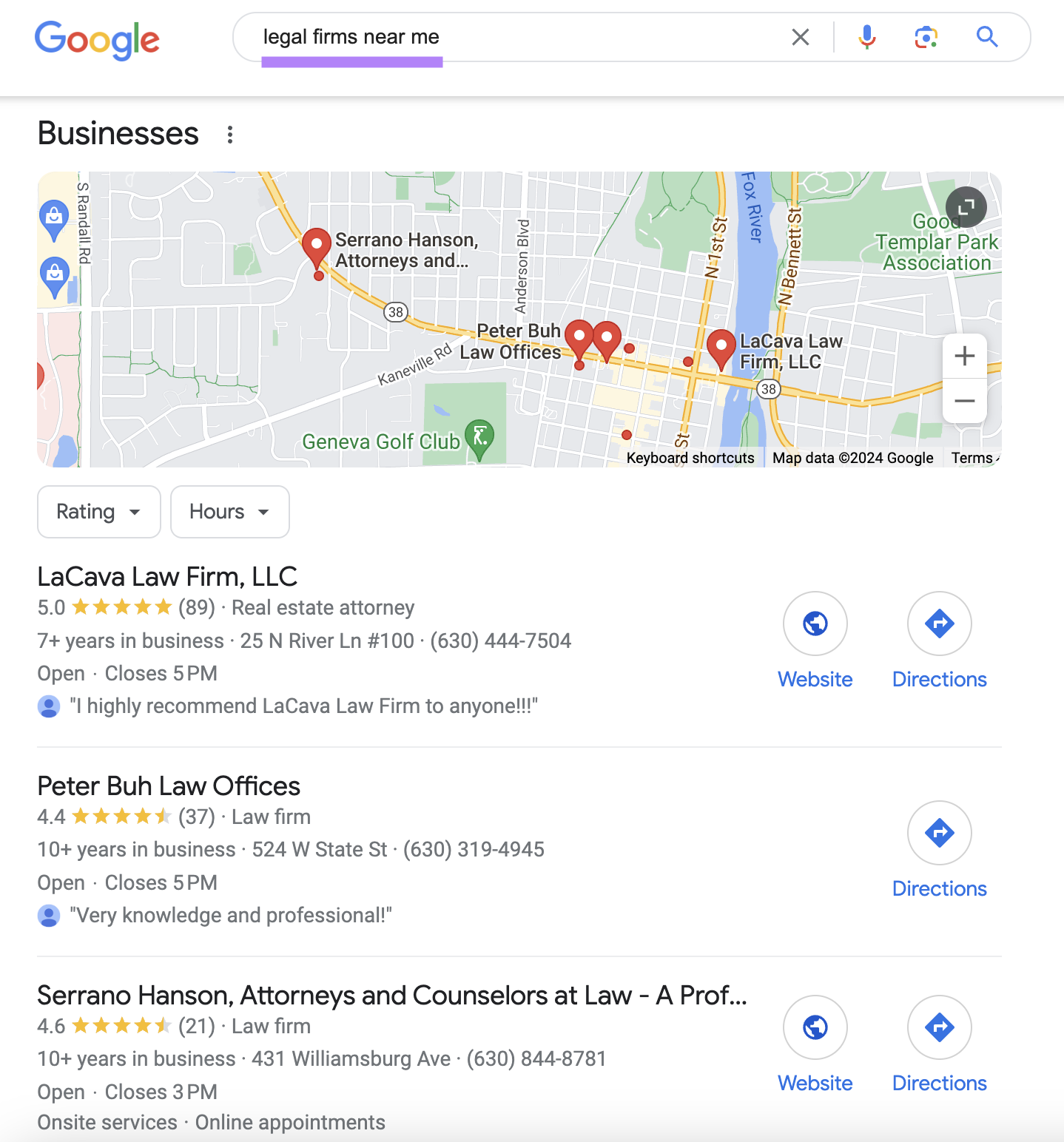The image is a screenshot of a Google search results page displayed on a computer screen. In the upper left corner, the colorful Google logo is prominently visible above a search bar, which contains the query "legal firms near me" highlighted in purple, indicating a previously clicked link. Below the Google logo, the word "Businesses" is displayed in bold black text.

Beneath this, a horizontally oriented rectangle map showcases various pinpointed legal firms. Several names are tagged on the map, accompanied by corresponding listings underneath. The top three listings include:

1. **La Cava Law Firm** – Operating for seven years, currently open, and closing at 5 PM.
2. **Peter Buch Law Offices (B-U-H)** – Rated 4.4 stars, in business for ten years, and also closes at 5 PM.
3. **Serrano Hanson, Attorneys and Counselors at Law, A Prof...** – Rated 4.6 stars, ten years in business, open now, but closes at 3 PM.

Additionally, the map indicates nearby locations such as Fox River and Geneva Golf Club, providing some geographical context, although the specific town remains unidentified. This detailed screenshot reflects a search for local legal firms in an unspecified area.